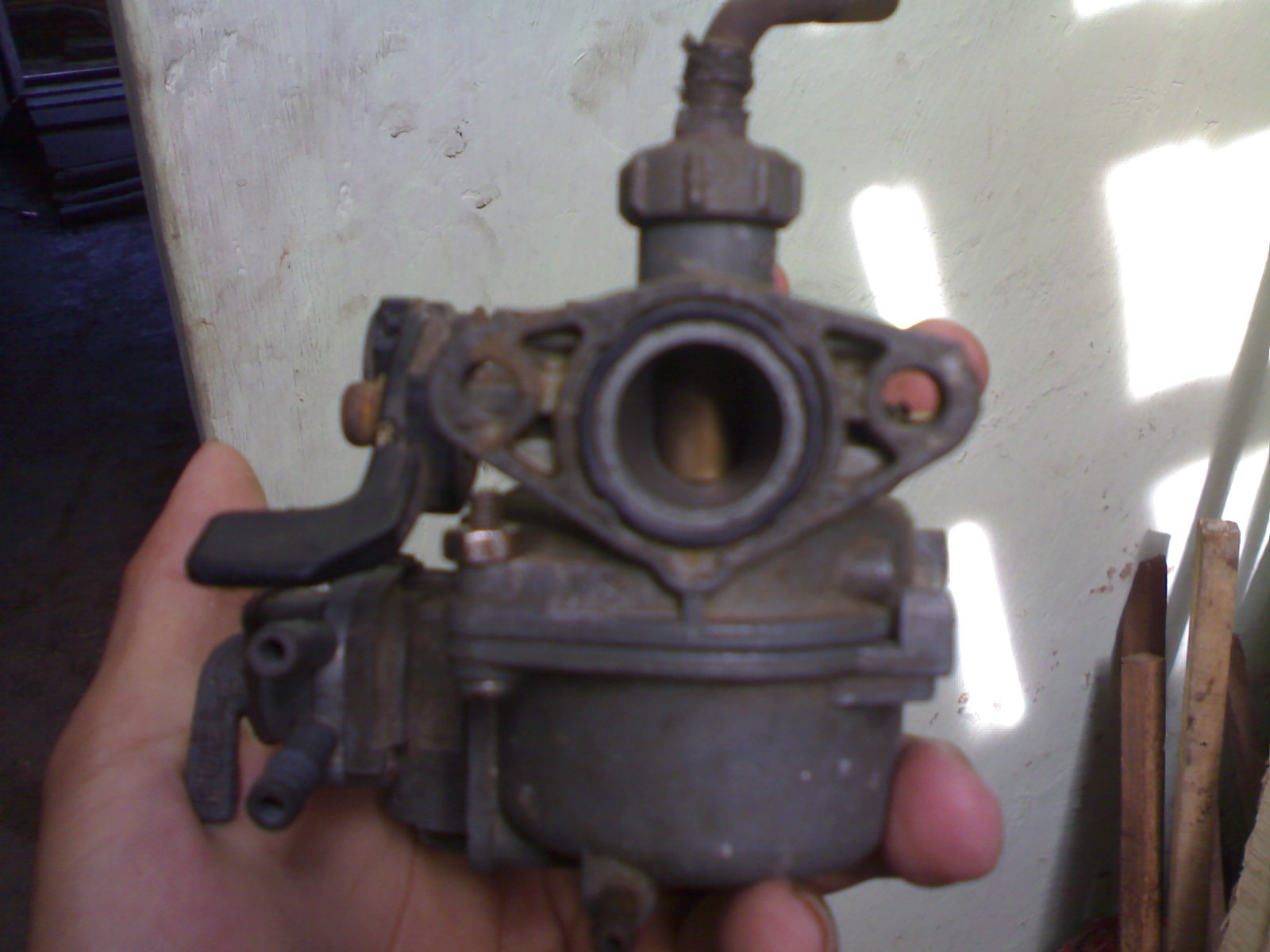The image depicts a close-up, vertical rectangular shot of a small automotive or mechanical part, resembling a pump, held in a white person's left hand. The background features a predominantly white wall with a light reflection on the right side and some wood leaned against it at the bottom right. Toward the upper left, there appears to be a gray-blue area, possibly a hallway.

The hand, slightly curved with palm up, reveals the thumb and fourth and fifth fingers, supporting the metallic, dark gray component in the center. The part is cylindrical and complex, with various openings, bolts, and protruding features, including a circular opening at the center top, akin to a fitting for a water hose, complete with ridges. Additionally, there is a smaller pipe sticking out from the top with a twist-on device. Various components, such as gears and perhaps a thumb lever, give the part a detailed, intricate structure.